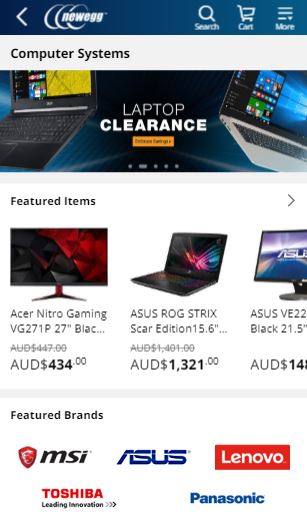In this image, we see a portrait-oriented screenshot, likely taken from a smartphone. This screenshot is from Newegg, an online retailer specializing in computer hardware and consumer electronics. The page displayed appears to focus on computer systems. At the top, there's a prominent banner labeled "Laptop Clearance," showcasing a few laptop models; users can click on either the laptops themselves or the banner to access the clearance section for laptops.

Below the banner, there is a "Featured Items" section, displaying three specific products. The first item is an Acer Nitro Gaming monitor, followed by an Asus ROG Strix Scar Edition laptop. The third item is another monitor, although the text is partially cut off. Notably, the prices of these products are shown in Australian Dollars (AUD), indicating that this is the Australian version of the site.

At the very bottom of the screenshot, there's a "Featured Brands" section highlighting several well-known brands including MSI, Asus, Lenovo, Toshiba, and Panasonic.